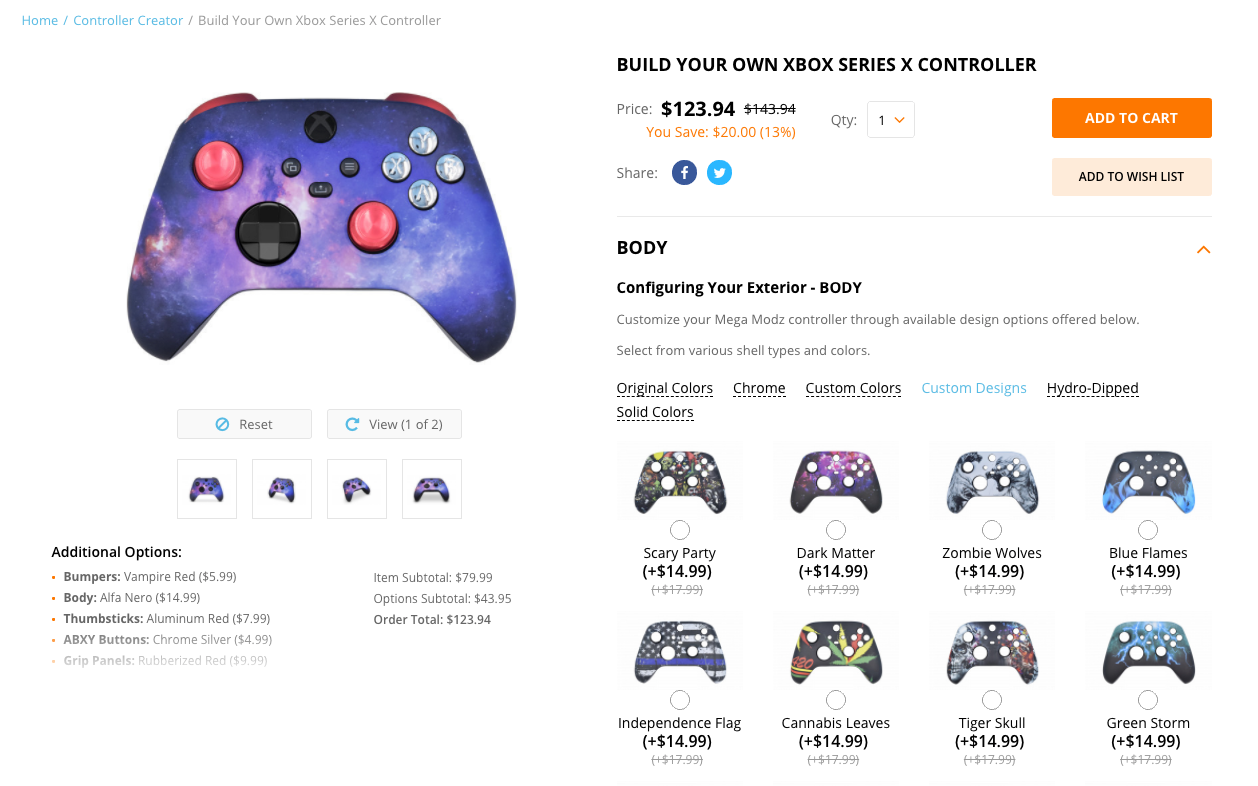This image is a screenshot from a webpage with a white background. In the upper left corner, it reads "Home / Controller Creator / Build Your Own Xbox Series X Controller." Below this heading is a photo of an Xbox Series X controller. The surface color of the controller features shades of blue and purple, resembling clouds. 

The controller's buttons are a mix of different colors: some are red, some are black, and four are silver. On the right side of the image, there is a headline that reads "Build Your Own Xbox Series Controller." The price is listed as $123.94, marked down from the original price of $143.94, indicating a discount. Beneath this, in orange text, it states, "You save $20 (13%)."

To the right of this text are two buttons. The first is an orange rectangle with white font that says "Add to Cart." Below it is a pink rectangle that says "Add to Wish List." Beneath these buttons, there are two rows of four controllers each, displayed with various background colors and images, giving users multiple customization options.

Above these rows, a headline states "Configuring Your Exterior," allowing users to select their desired controller design.